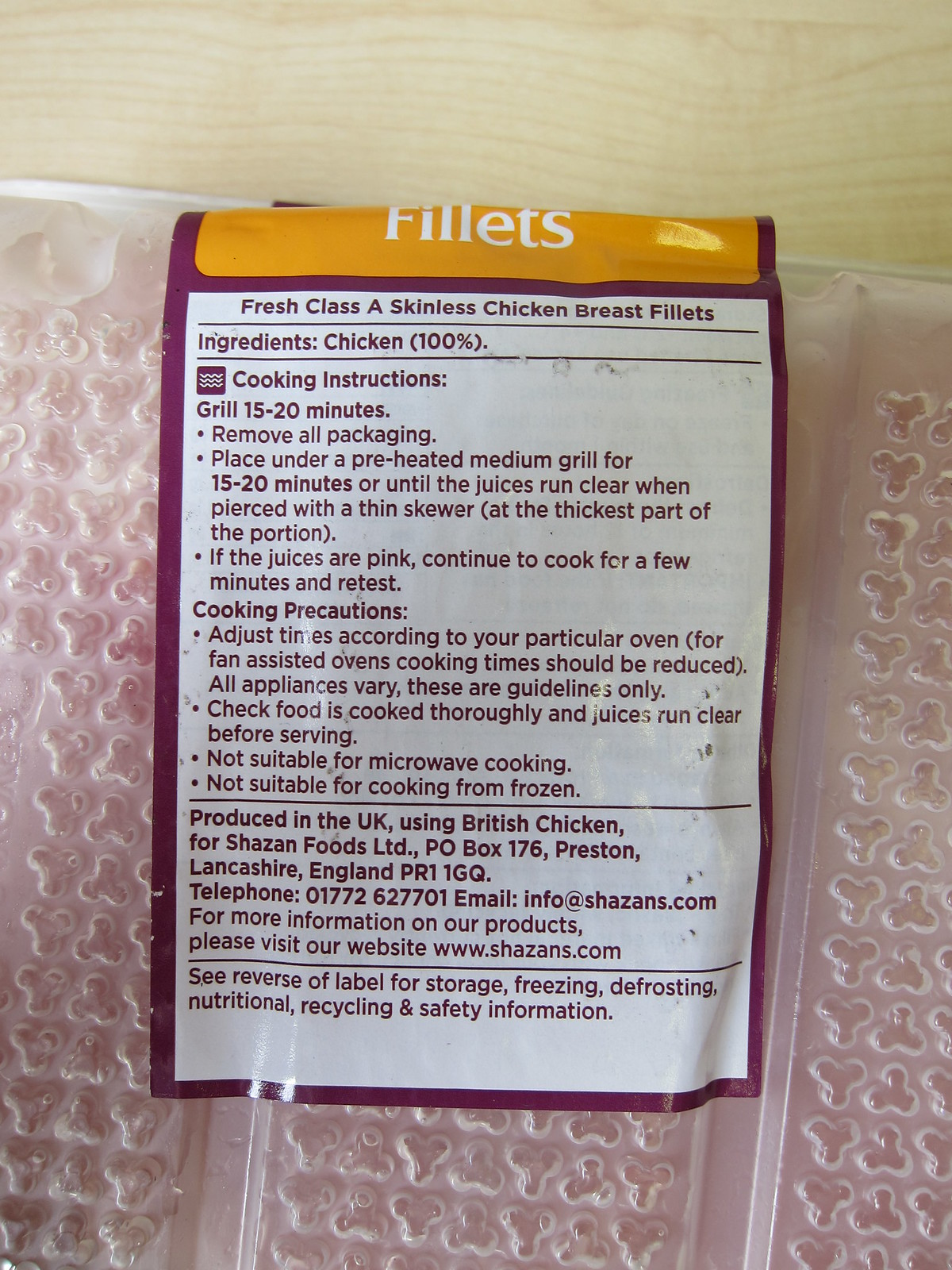The image showcases a prominently displayed package of fresh Class A skinless chicken breast fillets. The package, likely a plastic container, is set against a wooden surface, possibly a kitchen table or countertop, suggesting an indoor kitchen setting. The label on the package is predominantly maroon, with "fillets" written at the top in yellow against a white background. Key details visible on the label include the ingredients, which state "chicken 100%," and the cooking instructions. These instructions advise removing all packaging and grilling for 15-20 minutes on a preheated medium grill, ensuring that the juices run clear when pierced with a thin skewer at the thickest part. If the juices are pink, cooking should continue for a few more minutes and be retested. Additional information on storage, freezing, defrosting, nutrition, recycling, and safety can be found on the reverse of the label. The overall color palette of the image includes tan, brown, yellow, orange, maroon, and white, with the label prominently centered.